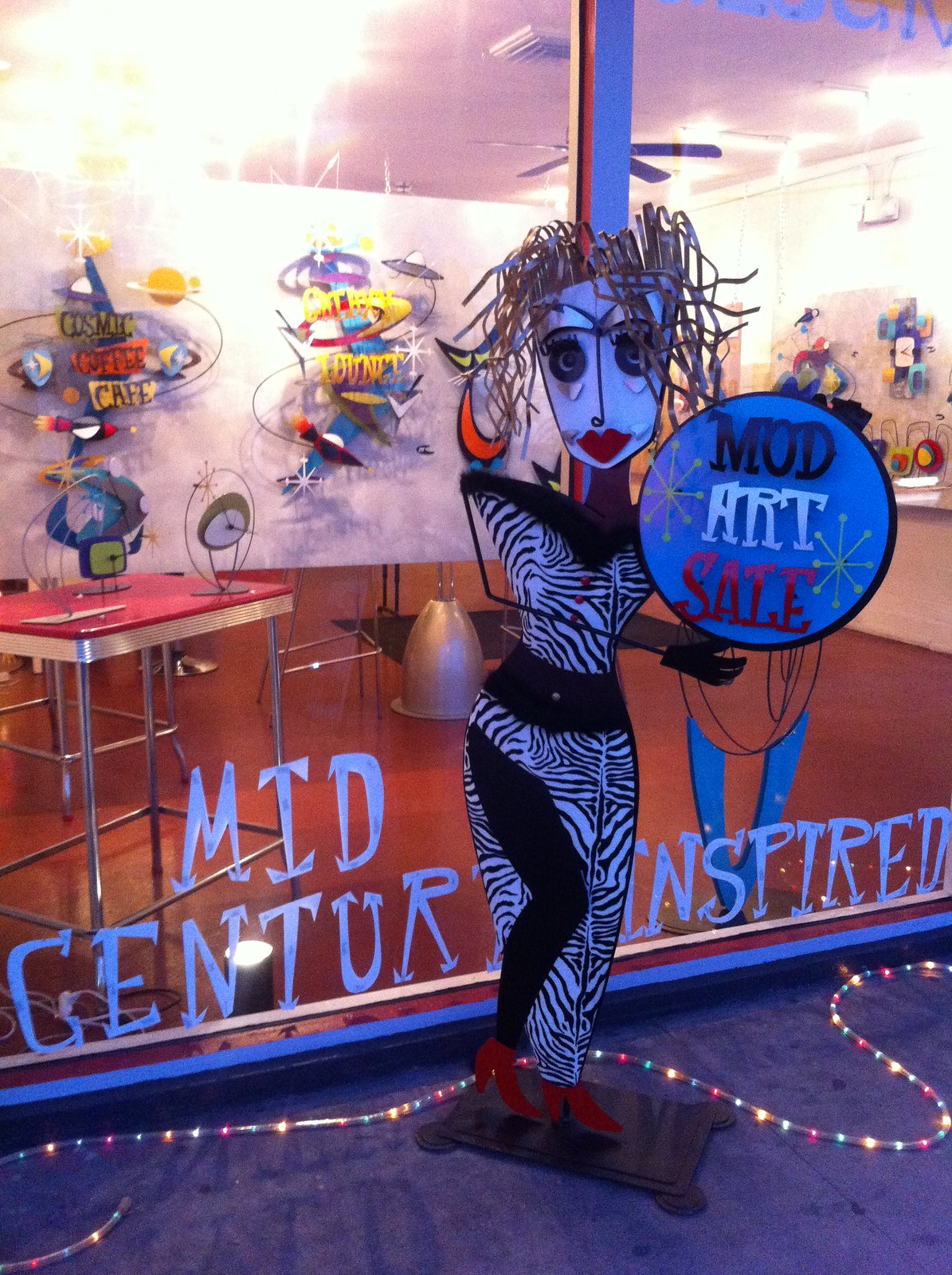The image features an eclectic storefront with a vibrant, artistic display. Central to the scene is an abstract sculpture of a human figure made from black metal rods and twisted copper strips for hair, resembling dreadlocks. This striking sculpture, with a cartoonish face made of iron rods, holds a sign that reads "Mod Art Sale." The ground surrounding the storefront is lined with LED lights, contributing to a colorful atmosphere. The window of the store displays the phrase "Mid-Century Inspired," hinting at the style of items sold within. Through the glass, one can see a variety of retro-inspired artistic pieces and sculptures arranged on a table, including two distinctive clocks. The interior is brightly lit, featuring colors like purple, yellow, green, blue, red, and pink, enhancing the abstract and inviting ambiance of this art store.